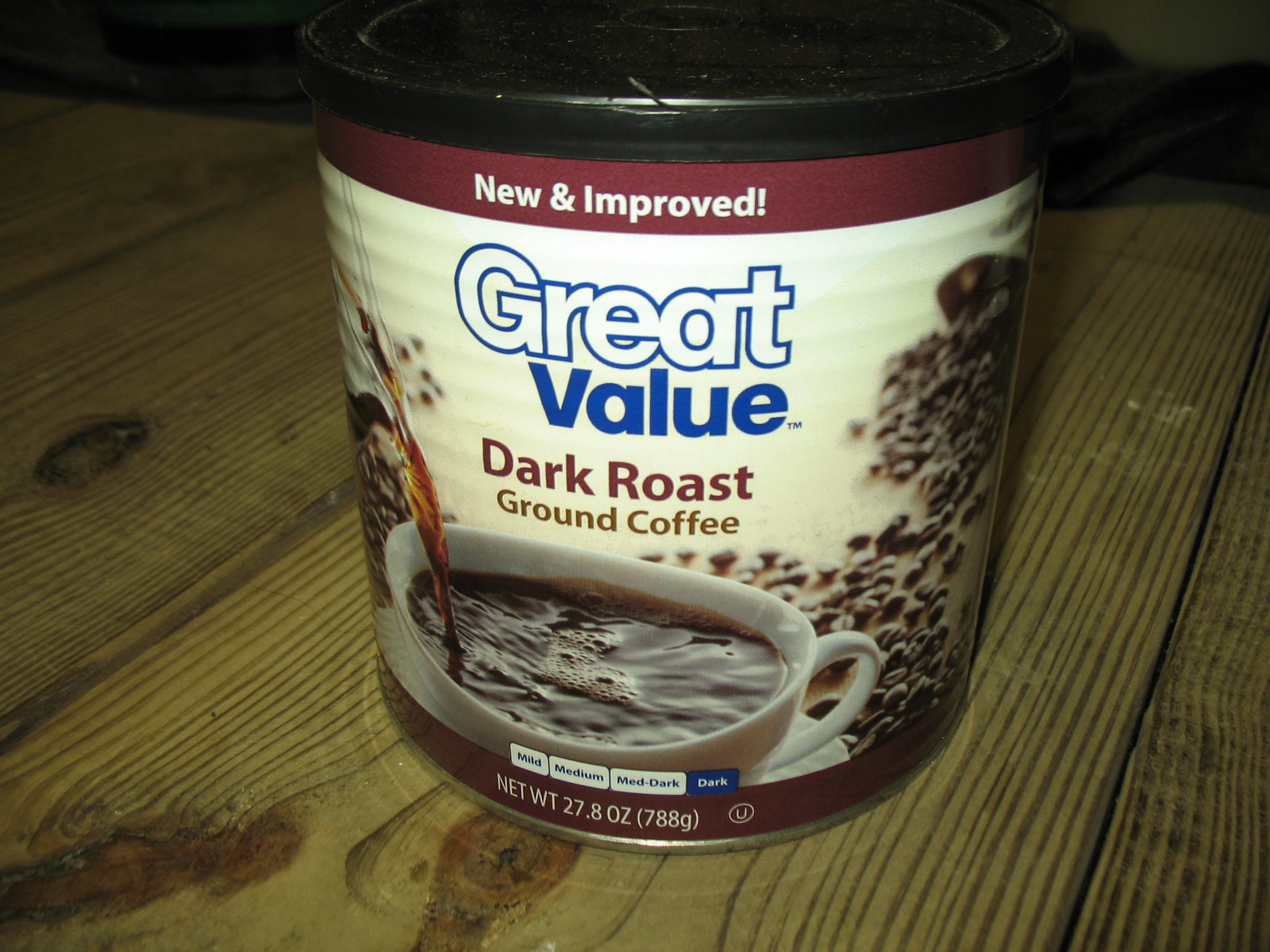This photograph captures a can of Great Value Dark Roast Coffee prominently displayed on a wooden surface. The label of the coffee can is a light tan hue, adorned with a detailed image of a white ceramic cup set on a matching saucer, with rich, dark brown coffee being freshly poured into it. In the background, scattered coffee beans are visible, spilling out of several open bags, adding texture and context to the scene. The can’s label also features two distinctive burgundy bands at the top and bottom, with white text that reads "New and Improved" at the top and denotes the net weight as "27.8 ounces" at the bottom. The overall ambiance of the photograph is somewhat dark and shadowy, contributing to a cozy, intimate atmosphere.